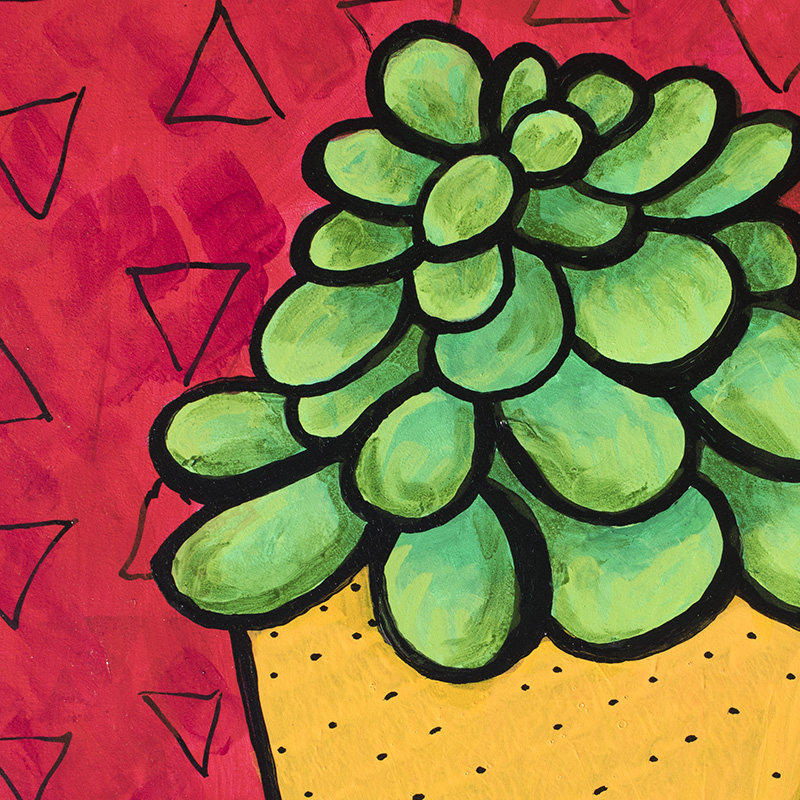The image is a cartoon-style painting featuring distinct shapes and vibrant colors. The background is primarily red, interspersed with darker red splotches and multiple black triangles oriented both upwards and downwards. Dominating the foreground on the bottom right is a square, yellow object resembling a sponge with numerous black dots and a black border. Atop this yellow form is a lush mound of rounded leaves, rendered in various shades of green, including light green, teal, and darker green accents. The leaves are also outlined with a thick black border, adding to the bold, whimsical style of the painting.